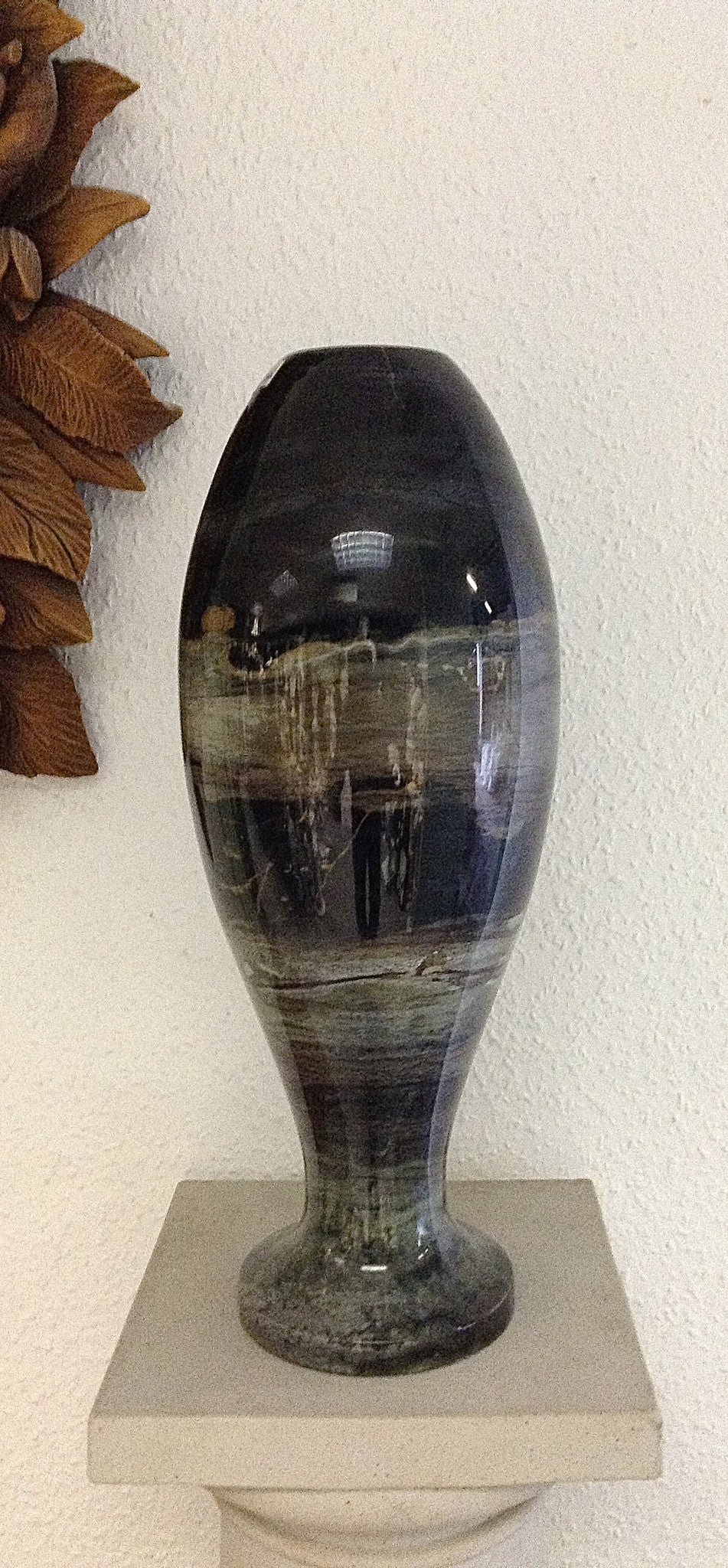The photograph features a striking vase-like art piece, potentially carved from a highly reflective stone, resembling granite. Its distinctive shape, reminiscent of an inverted bowling pin, includes a roundish base that flares out, narrows in the middle, and then flares out again before tapering towards the top. The surface is predominantly black with elegant gray stripes running through it, enhancing its polished appearance. The vase rests on a simple, white or light gray marble pillar that has a round shape with a square cap.

The background consists of a white stucco wall, flatly lit, adorned with decorative, carved wooden leaves to the left, which appear brown and may be either real or artificial. Details within the room emerge in the vase’s reflection, with visible figures that seem to include a man in a suit and a chandelier overhead. The intricate interplay of reflections and ambient decor adds an additional layer of depth to the already intriguing composition.